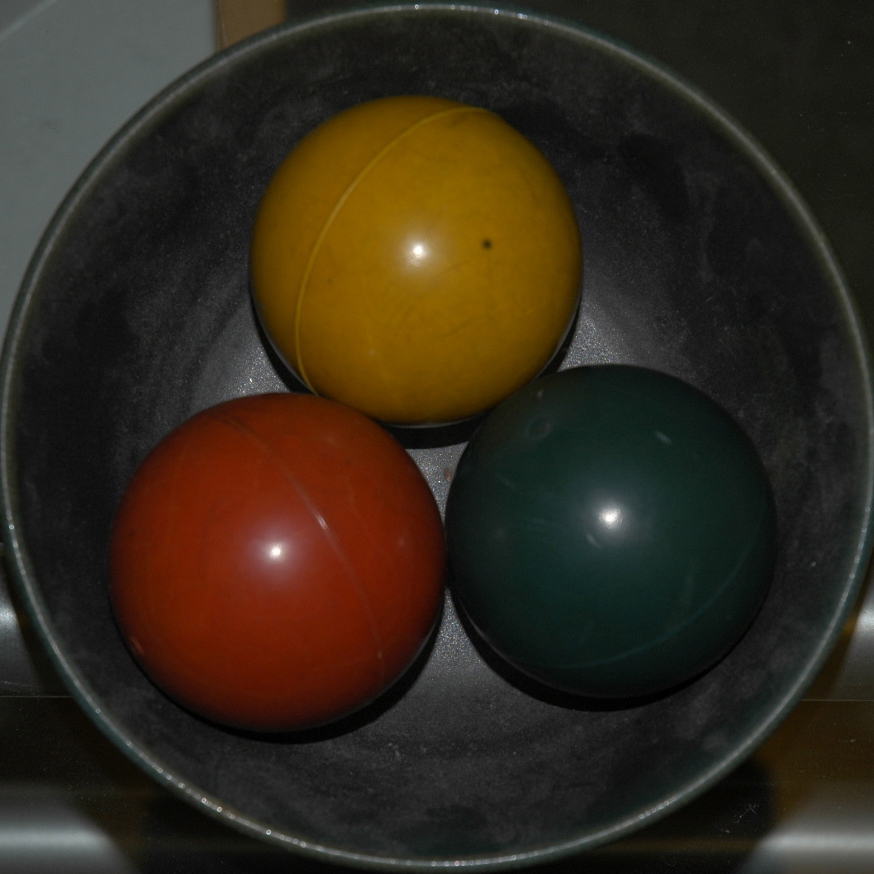This square image, viewed from directly overhead, captures a grayish bowl, potentially made of ceramic or cast iron, occupying 90% of the frame. The bowl is smooth, with no distinct features except for a reflection of a ceiling lightbulb, hinting at the image's dark ambiance. Inside the bowl are three heavy, smooth, baseball-sized balls with clear seams around their middle. The balls, reminiscent of traditional wooden croquet balls, are positioned as follows: a red ball in the bottom left, a dark green ball in the bottom right, and a yellow-golden ball at the top middle. The image background is blurry, offering no additional context about their exact material or purpose.